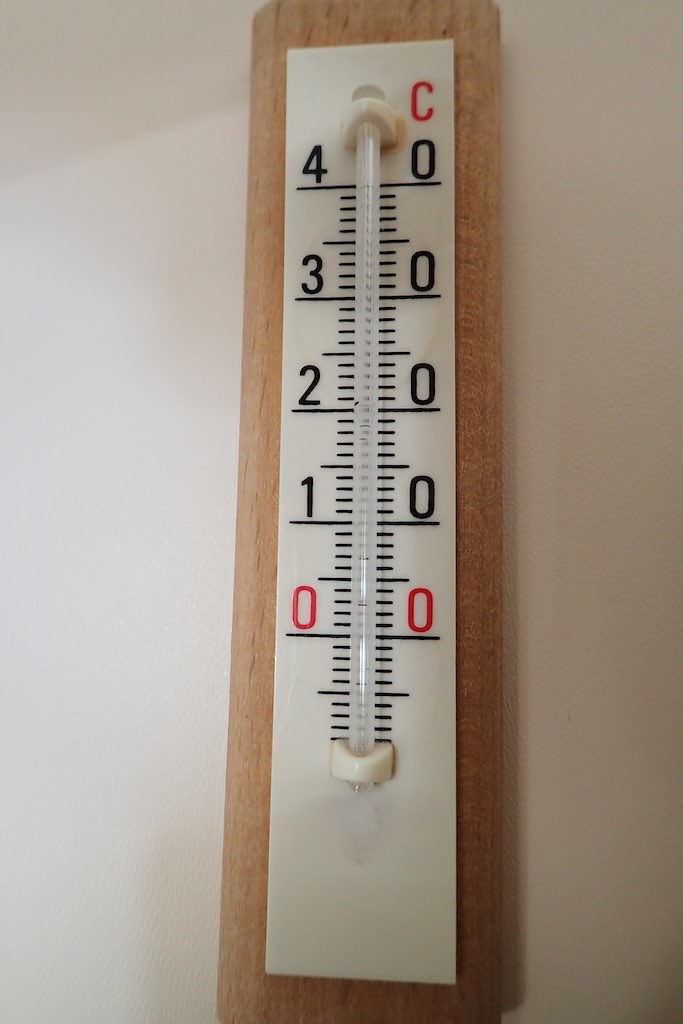This image features a vintage thermometer with a long, rectangular white base. In the top right corner, a prominent red capital "C" marks the Celsius scale. A clear cylindrical tube runs down the length of the thermometer, extending from the top of the numbered scale to the bottom. The numbers on the scale are arranged in descending order, starting with "40" on the left side. The bold black "40" is paired with a "0" on the right, and this pattern repeats down to "30", "20", and finally to "0". At the "0" mark, the font color shifts from black to red, signifying a key point in the scale.

Each number is aligned with a thick black line, and between these main markers are smaller lines. These medium black lines appear in the center between each set of numbers, providing more precise gradations. Thinner black lines further subdivide the scale for even finer measurement.

The thermometer is secured at both ends by beige brackets that hold it in place, ensuring accurate readings. This unit is mounted on a medium-brown piece of plywood, which shows slight variations in shade—darker on the right, possibly due to shadowing.

The entire setup is affixed to an off-white wall, typical of industrial settings. The wall's texture is visible, characterized by small dots and lines, especially noticeable in the bottom left corner, suggesting a tactile, slightly rough surface.